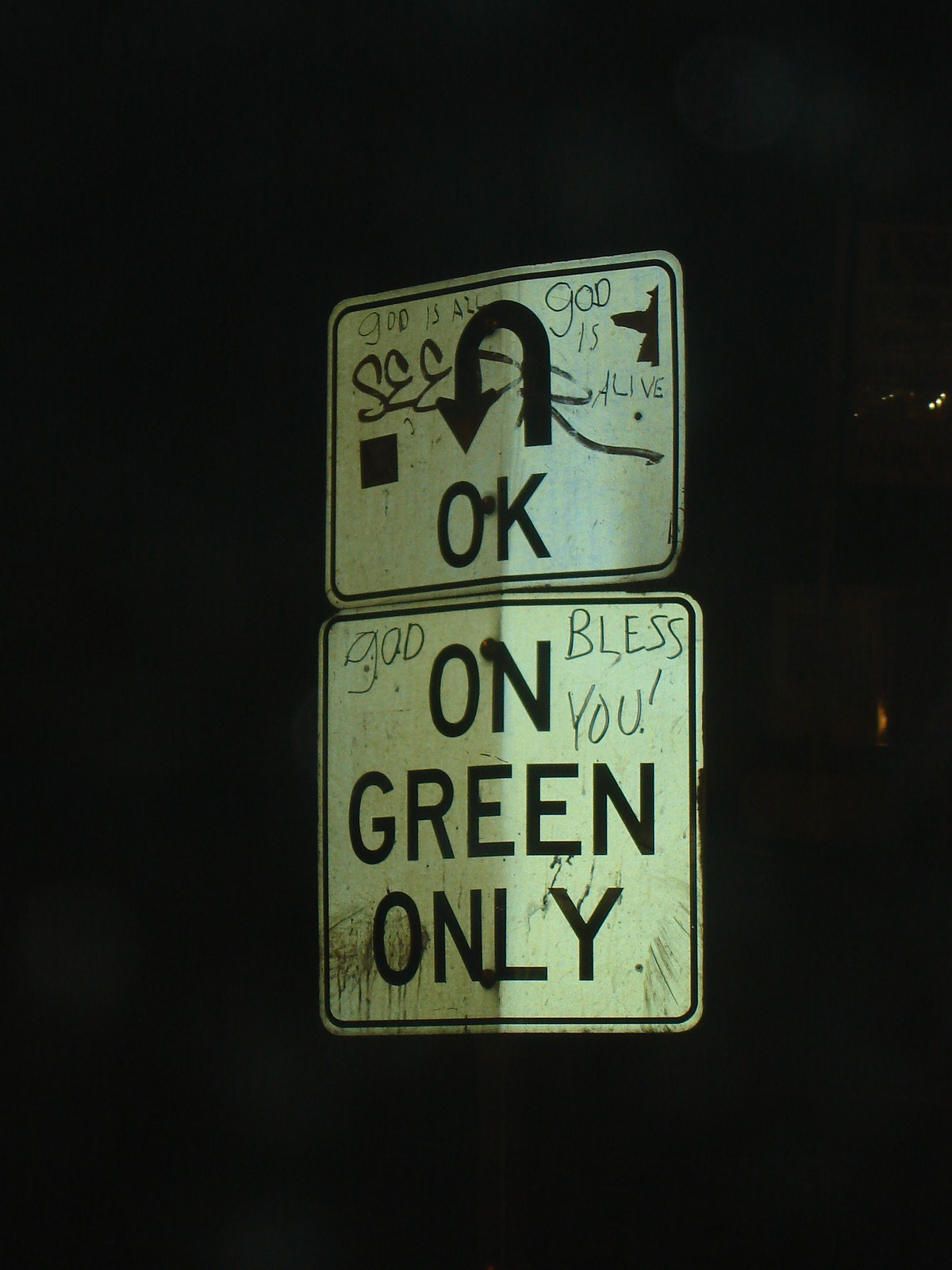This photograph captures two road signs against a pitch-black night sky, casting them in shadow. The signs, both square and white with black text, are riddled with graffiti. The top sign features a U-turn symbol followed by the word "OK." Scrawled across this sign in black marker are the phrases "GOD IS ALL," "GOD IS ALIVE," and "GOD IS LIFE," along with the word "SEER." The bottom sign, slightly larger, instructs "ON GREEN ONLY" in black text. It too bears graffiti, with "BLESS YOU" written beside the official text, and "GOD" scribbled to the left. Dark drips of a liquid, possibly thrown, streak down, further distorting the surface. The night enshrouds the signs, making the writings stand out starkly against the whiteness.